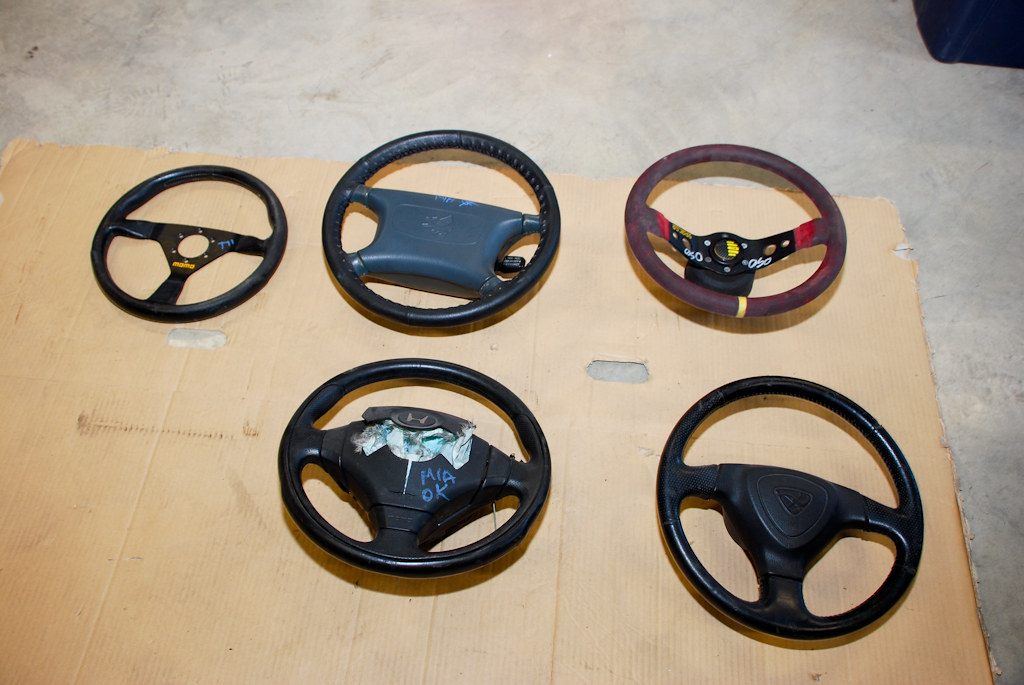This rectangular photograph showcases five steering wheels arranged on a piece of cardboard, which is placed on a gray concrete floor. The cardboard sheet is incomplete, cutting off on the left side. The top row features three steering wheels: the one on the far left is black and the smallest, the middle one is slightly larger and also black with a gray center, and the steering wheel on the right is dark purple with a red and black center adorned with a yellow knob. The bottom row presents two more black steering wheels; the left one has an "H" emblem suggestive of a Honda, accompanied by the blue handwritten text "MIA OK" and some golden accents in the center, while the right one is a simple black steering wheel.